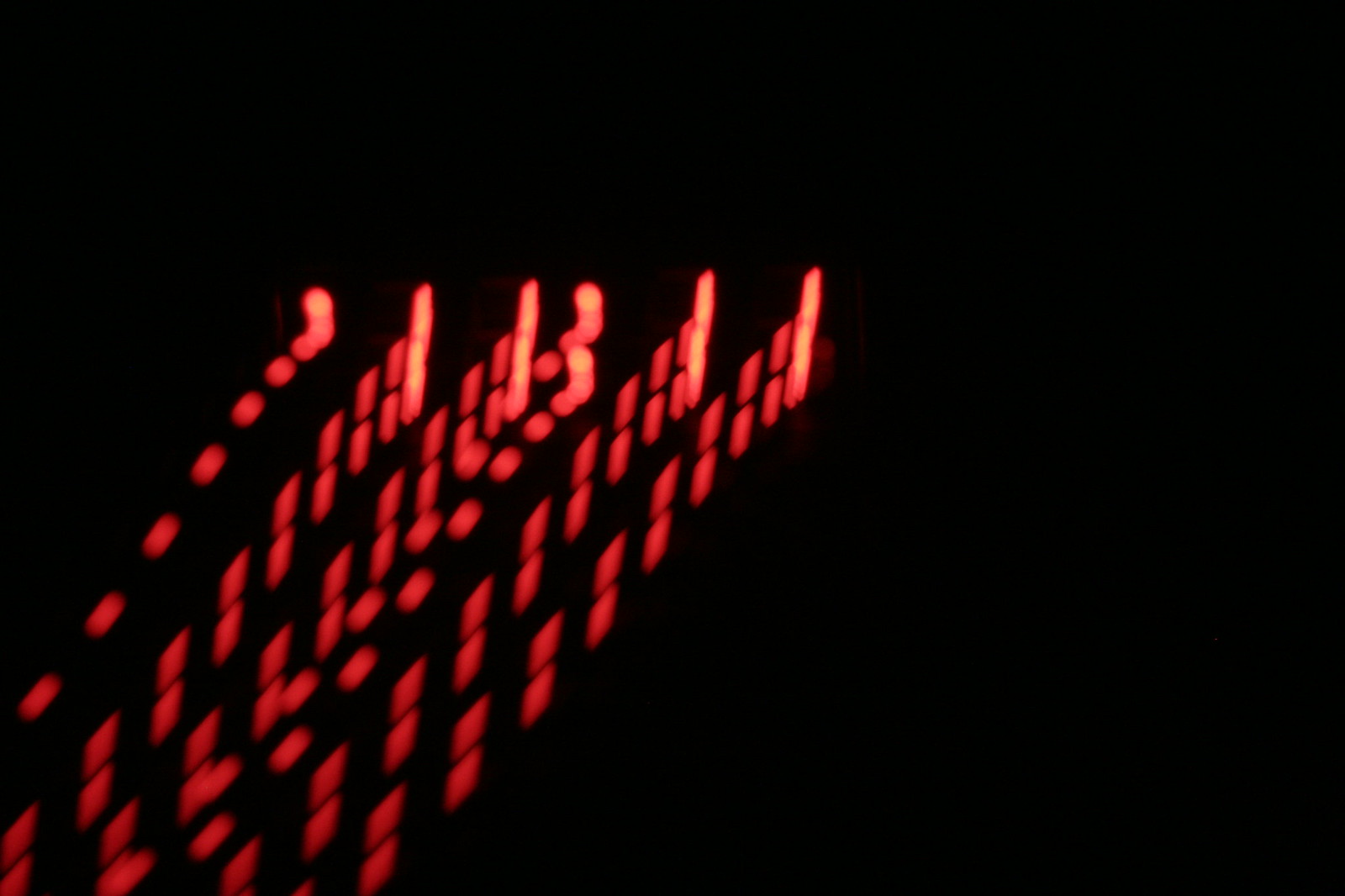A stark image dominated by a pitch-black background features a striking pattern of streaky red lights. The central focus of this composition is an array of six elongated rows of red LED-like illumination, resembling the hex digits seen on a digital clock but dragged sideways, creating the illusion of a tar tread. Each row contains both single and double dots, trailing diagonally from the center-left towards the lower left corner. These dots, which blur and fade as they extend, evoke the impression of neon lights in motion, perhaps captured with a slow shutter speed. The vivid red light disrupts the complete darkness, casting an almost futuristic, hypnotic effect across the image.